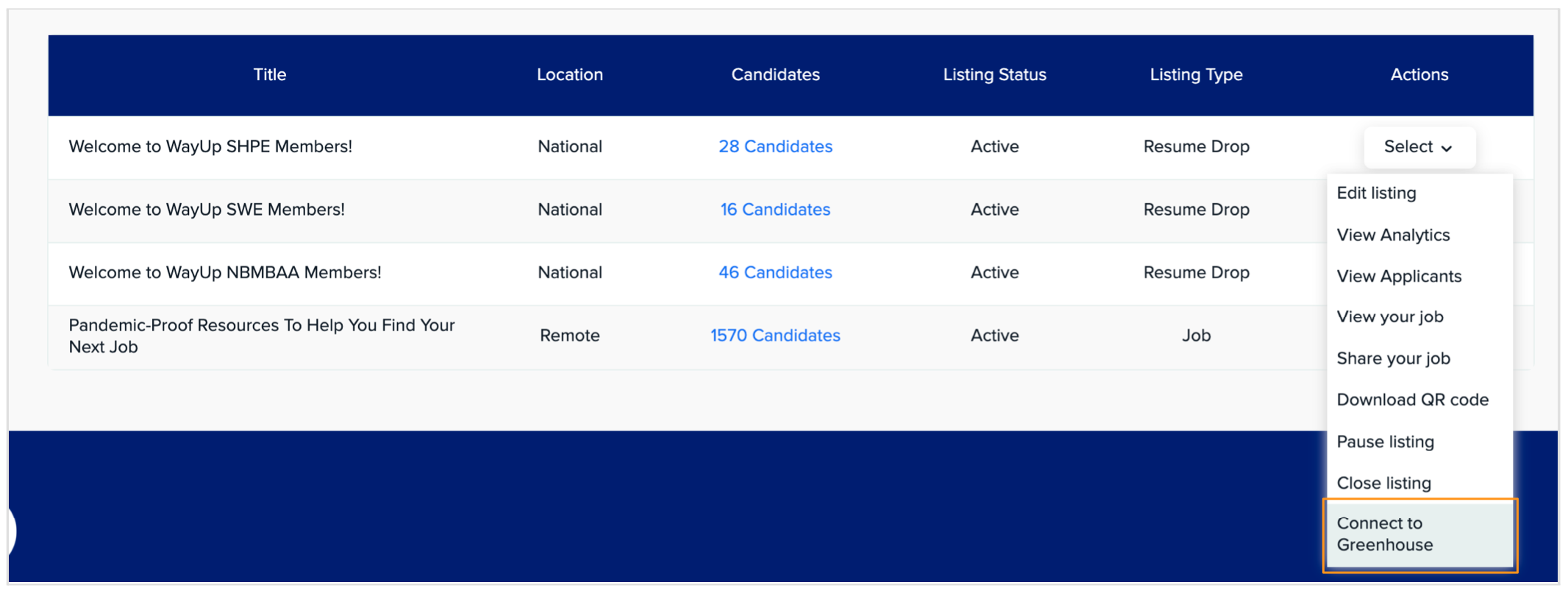This is a detailed screenshot of a website interface showcasing a spreadsheet-style layout with a navy blue header bar labeled with white text. The columns are titled:

- Title
- Location
- Candidates
- Listing Status
- Listing Type
- Actions

Below the "Title" column, the entries are:
- "Welcome to Weyup SHPE members"
- "Welcome to Weyup SWE members"
- "Welcome to Weyup NBMBAA members"
- "Pandemic Proof Resources to help you find your next job."

Under the "Location" column, the entries are:
- "National"
- "National"
- "National"
- "Remote."

In the "Candidates" column, the entries are:
- "28 candidates"
- "16 candidates"
- "46 candidates"
- "1,570 candidates."

The "Listing Status" column shows "Active" for all entries. 

The "Listing Type" column includes "Resume Drop" for the first three entries and "Job" for the last entry.

To the right, under the "Actions" column, a drop-down menu labeled "Select" is open. This white square menu contains the options:
- "Edit Listing"
- "View Analytics"
- "View Applicants"
- "View Your Job"
- "Share Your Job."

This comprehensive screenshot provides a well-structured view of various job listings and their pertinent details, making it easy to manage and analyze each entry.